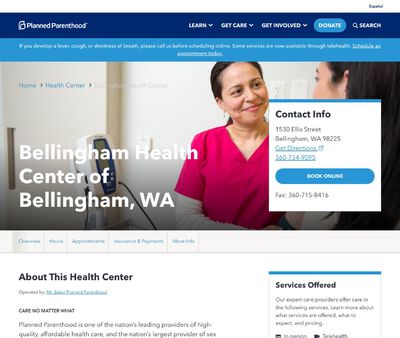This is a detailed screenshot of the Planned Parenthood website. At the top, there is a prominent blue banner displaying the organization's name, "Planned Parenthood." Below the banner, there's a navigation menu with dropdown options such as "Learn," "Get Care," and "Get Involved," alongside a "Donate" button and a search icon resembling an hourglass with the text "Search" next to it.

Just beneath this, a lighter blue banner with difficult-to-read white font advises visitors to call in advance if they are experiencing symptoms like cough or shortness of breath before scheduling an appointment.

Lower down the page, taking up most of the screen, is a large image showing two women engaging with each other. Overlaid on the image are red crowns and partially readable text that includes "Health Center" and "Bellingham" in white font. Near the bottom, the text clearly reads "Bellingham Health Center of Bellingham."

To the right side of the image, there is a contact form with a prominent blue button labeled "Book Online," accompanied by some contact information.